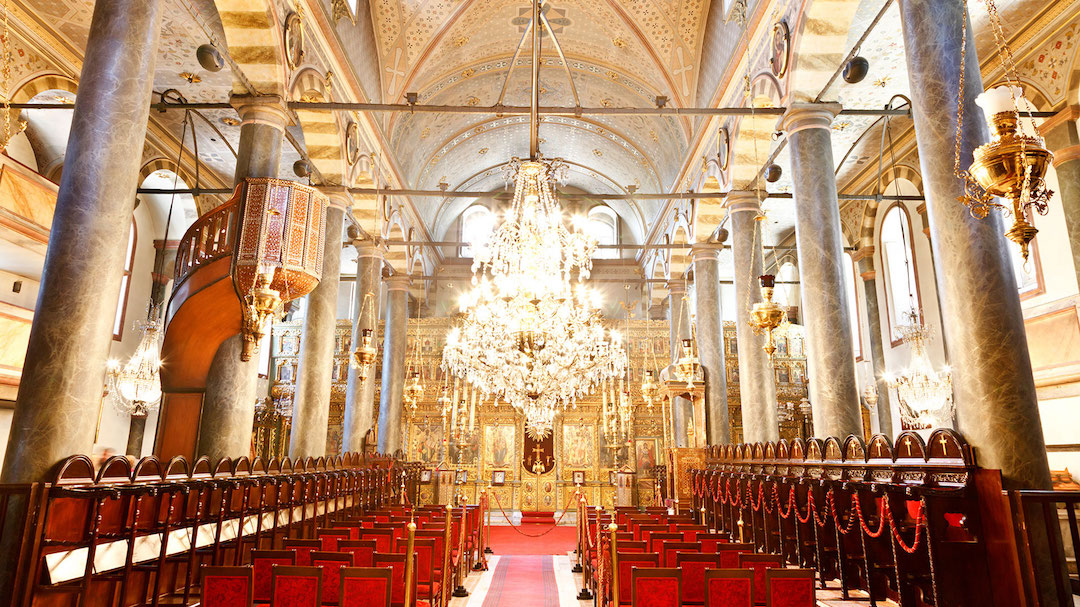The image depicts the stunning interior of a historically significant church, adorned with intricate Greek-style architectural elements. A massive glass chandelier dominates the center, casting a warm glow over the spacious nave. The church features a unique minaret that has been repurposed as a bell tower, blending different cultural influences seamlessly. A prominent symbol of Christ is displayed at the far back, serving as the focal point of the worship space. Rows of chairs are meticulously arranged in the center, inviting congregants to sit and reflect.

The walls are adorned with an elaborate mosaic pattern, interspersed with various suspended crosses that add to the spiritual ambiance. The marble flooring and towering marble pillars on either side enhance the grandeur of the interior. Given the exquisite craftsmanship and architectural splendor, this church is likely of great historical and cultural value. The pristine condition suggests it has recently opened to the public, ready to welcome visitors and worshippers alike.